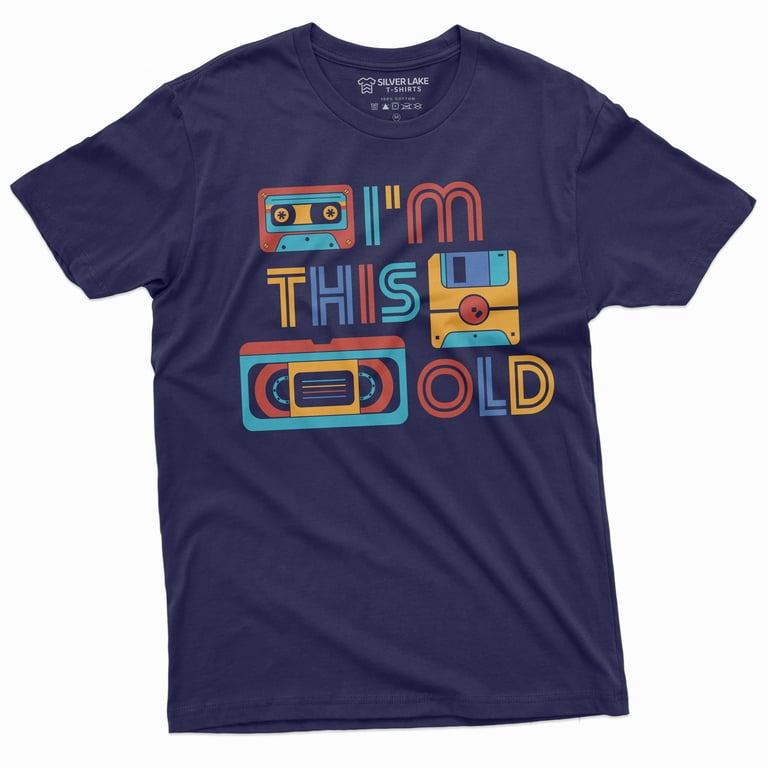This is a navy blue, short-sleeve crewneck t-shirt made by Silver Lake T-Shirts, in a likely medium size. The front of the shirt displays the phrase "I'm this old" in a retro design, with each letter in a different color, primarily teal, orange, and yellow. Above the phrase is an image of an orange and teal cassette tape, and following the words "I'm this" are images of a floppy disk and a VHS tape, all in varying shades of orange, yellow, and teal, creating a nostalgic 80s and 90s aesthetic. The font is entirely capital letters, with some letters mimicking styles like the McDonald's arches for the "M" and double letters for an added retro effect. The background of the image is plain white, highlighting the vibrant colors and intricate design details of the t-shirt.